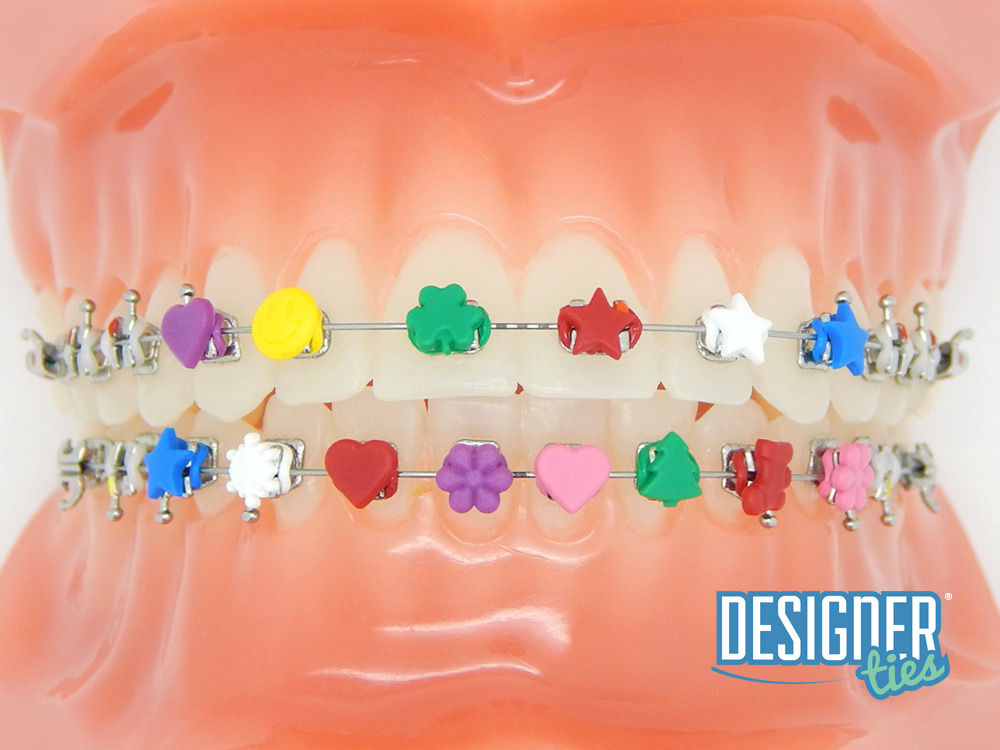This image depicts a detailed model of an orthodontic set designed to showcase decorative braces. The model features both upper and lower artificial teeth, prominently displayed with flesh-toned, shiny gum molds. Each row of teeth is fitted with silver wires akin to traditional braces, adorned with a variety of colorful charms and decorations. 

On the top row, from left to right, the sequence of charms includes a purple heart, a yellow circle, a green clover, a red star, a white star, and a blue star, followed by three additional silver brackets. The bottom row is similarly embellished with a blue star, a white snowflake, a red heart, a purple flower, a pink heart, a green tree, a red stocking, a red teddy bear, and a pink teddy bear, interspersed with silver pieces. 

In the bottom right corner of the image, there is a logo with the word "designer" in white letters, outlined in blue, and beneath it, the word "ties" in a green script with a blue outline, further highlighted by a white circled “R” symbolizing a trademark. The overall presentation lends a festive and stylish appeal to the orthodontic accessories, emphasizing the designer's eye-catching and colorful options for braces decorations.